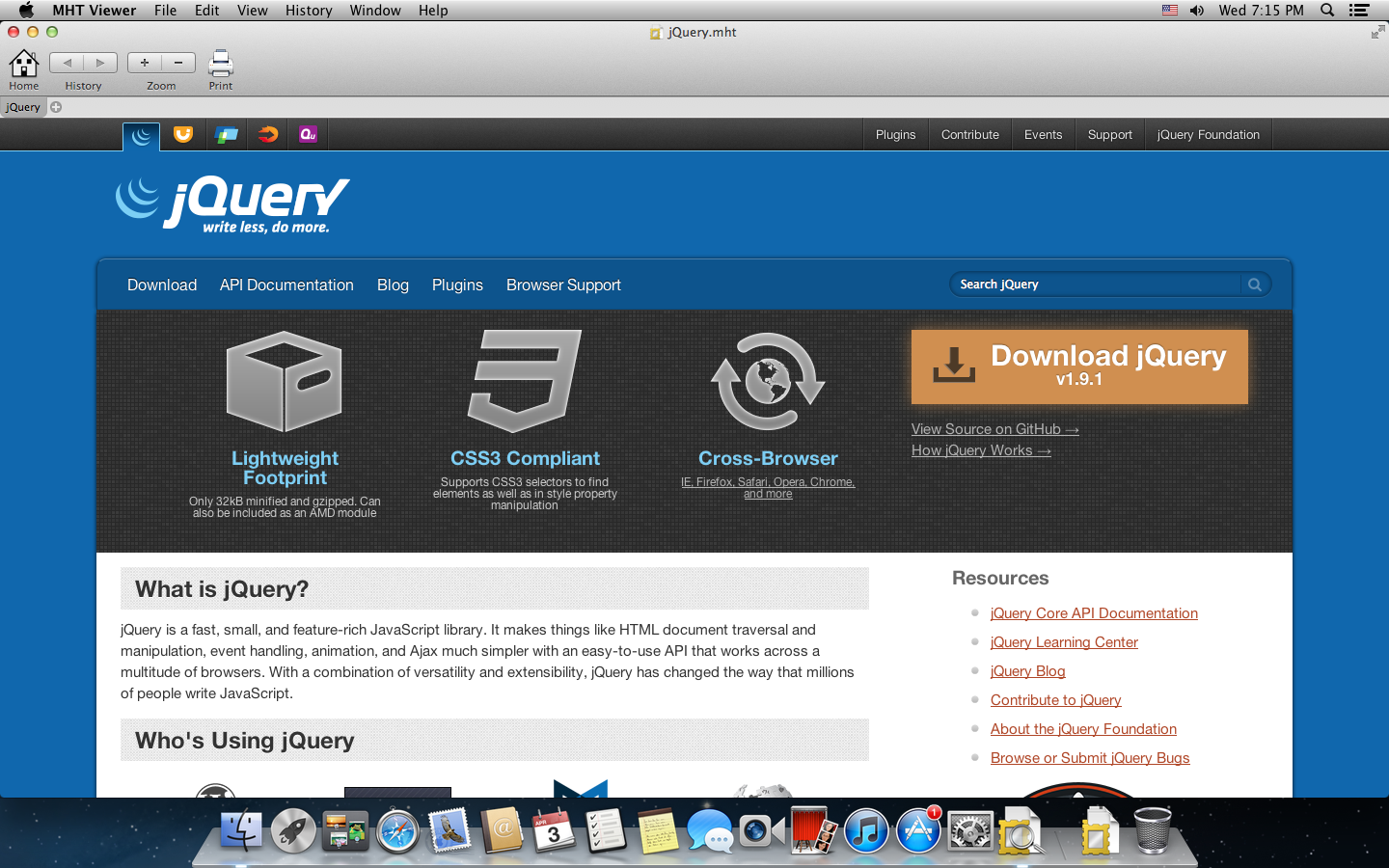The image depicts a Mac displaying a website in a browser window. In the top-left corner of the screen, the recognizable Apple icon confirms the operating system. The browser interface shows several menu options including "File," "Edit," "View," "History," "Window," and "Help." Towards the top right, symbols such as an American flag, a speaker icon, and a magnifying glass are visible, along with the time, which reads 7:15 PM on a Wednesday. Another icon featuring black horizontal lines is also present, albeit unclear.

Below this interface is the main browser window, featuring the jQuery website. The familiar red, yellow, and green buttons for closing and minimizing windows are located in the top-left corner. The website itself boasts a primary blue background. At the very top, a gray horizontal navigation bar spans the width of the page, featuring multicolored icons—blue, orange, blue, red, and purple—on the left side. On the right side of the bar, links to "Plugins," "Contribute," "Events," "Support," and "jQuery Foundation" are neatly aligned.

Prominently displayed in the main section, the jQuery tagline "Write Less, Do More" is highlighted. Below this, in white text, are links for "Download," "API Documentation," "Blog," "Plugins," and "Browser Support." Adjacent to these links is a search box. The central part of the webpage contains a noteworthy orange rectangular box with details about downloading jQuery. This section is complemented by icons and text for "Lightweight Footprint," "CSS3 Compliant," and "Cross Browser" in light blue, with accompanying gray icons above each text block.

Overall, the detailed elements and the clear layout contribute to a comprehensive and user-friendly interface.